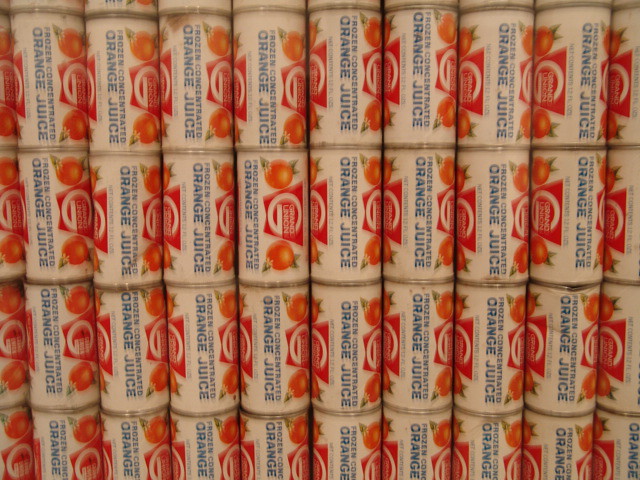The image captures several rows of orange juice containers, specifically frozen concentrate in white cans. These containers are oriented in various directions, making it challenging to read the labels clearly. Each can features a design that repeats around the entire container. 

In the top left corner of each label, there is an image of an orange, accompanied by some green leaves. The center of the label has a prominent white "G" against a red background. To the right, another orange appears, and beneath it, the words "frozen concentrate" are written in blue text. Below that, in larger blue letters, the label reads "orange juice." 

The cans are stacked in columns; the topmost visible layer shows ten cans per column with four columns in total, summing up to forty cans on the top level. The pattern continues in the lower levels, though the bottom cans are slightly cut off, displaying only part of their labels.